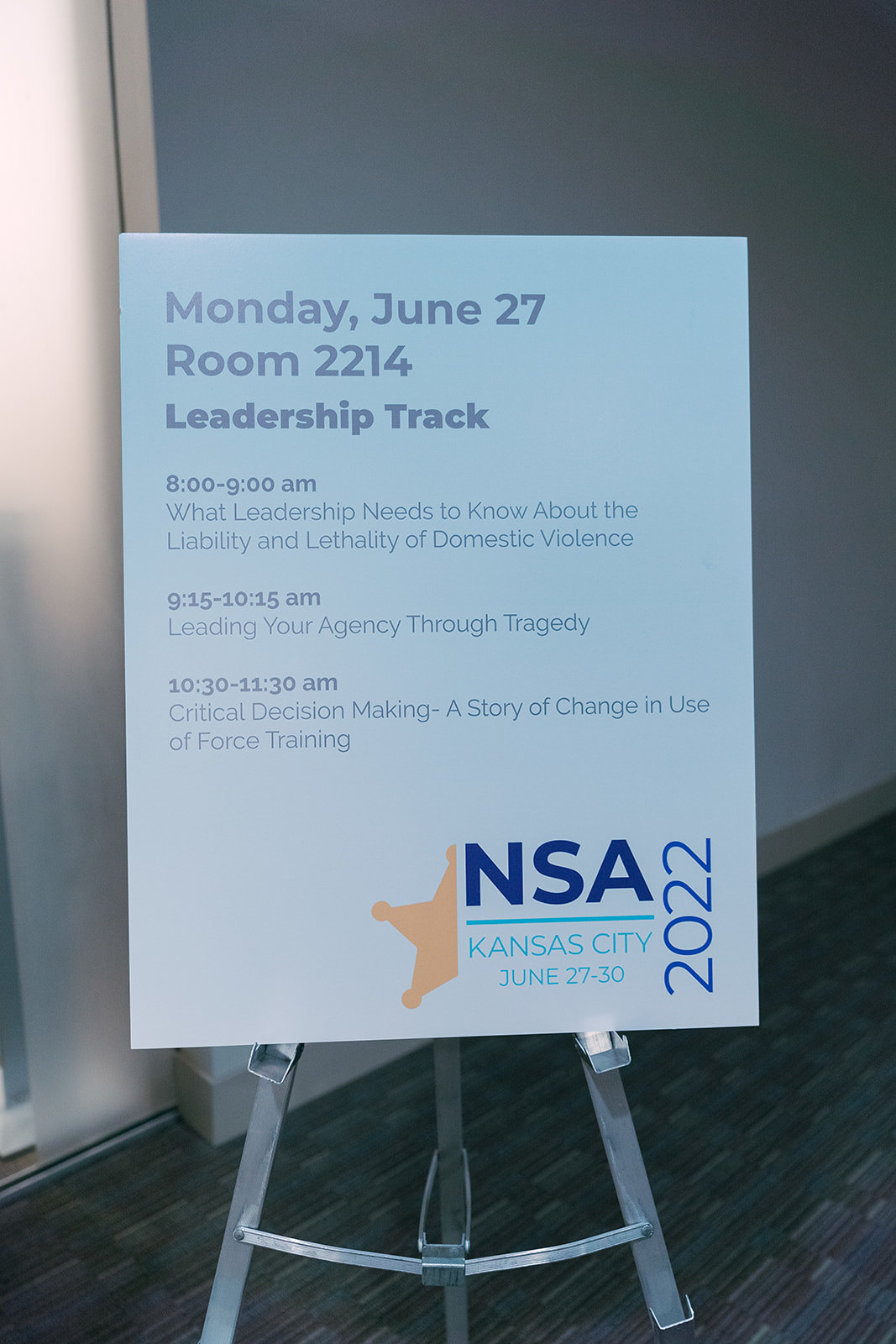This image captures a detailed sign set on a metal easel in a hallway, with a wall behind it, likely outside a conference or meeting room. The sign is white with blue text and outlines the schedule for a series of leadership lectures. The header reads: 

"Monday, June 27th, Room 2214, Leadership Track." 

Beneath this, the schedule is listed:
- **8:00 to 9:00 a.m.**: "What Leadership Needs to Know About the Liability and Lethality of Domestic Violence."
- **9:15 to 10:15 a.m.**: "Leading Your Agency Through Tragedy."
- **10:30 to 11:30 a.m.**: "Critical Decision-Making: A Story of Change in Use of Force Training."

The bottom right of the sign displays the text "NSA" in blue, alongside a small gold badge to the left. Below this, an aqua-colored text reads: "Kansas City, June 27th through 30th, 2022."